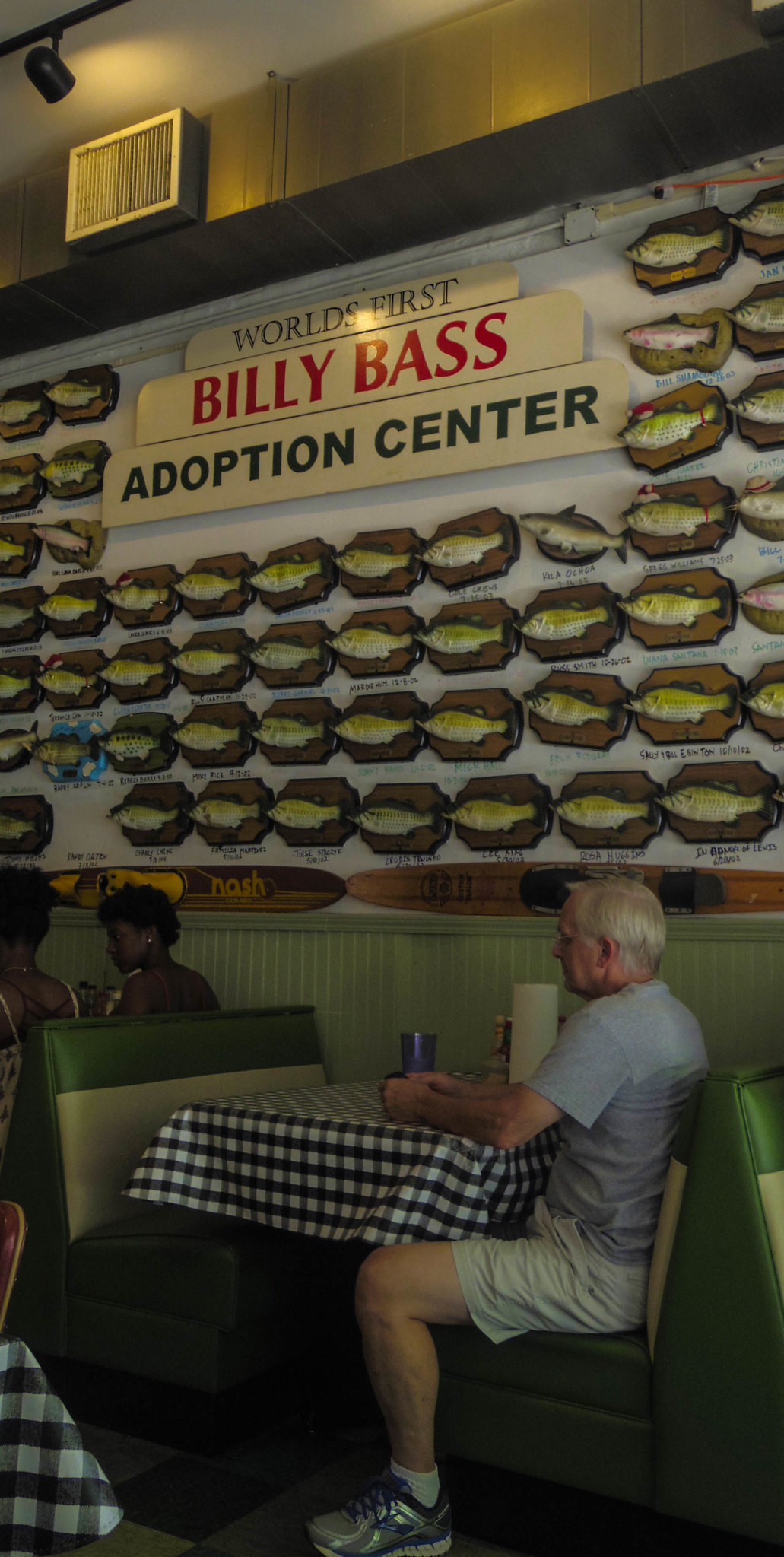The photograph captures a detailed scene inside a restaurant, focusing on a unique wall display that reads "World's First Billy Bass Adoption Center" in red lettering. The wall is densely adorned with wooden plaques, each mounting a yellow-gold singing Billy Bass fish, creating a vibrant backdrop. Below this, two wooden water skis are also mounted, adding to the eclectic décor. The setting includes several booths with green seats and black and white checkerboard oilcloth tabletops. 

In the lower right corner, a man with white hair is seated at a table covered with a blue and white checkered tablecloth. He is dressed in a short-sleeved gray t-shirt, light gray shorts, and gray running shoes. His table holds a roll of paper towels and a purple cup. He appears to be facing to the left, with his arms resting on the table, and he's the only one at his booth.

Adjacent to this man are two black women with short curly hair, seated in a booth to his left and engaged in conversation. The detailed décor and engaging human elements create a vibrant and lively atmosphere in the depicted restaurant scene.